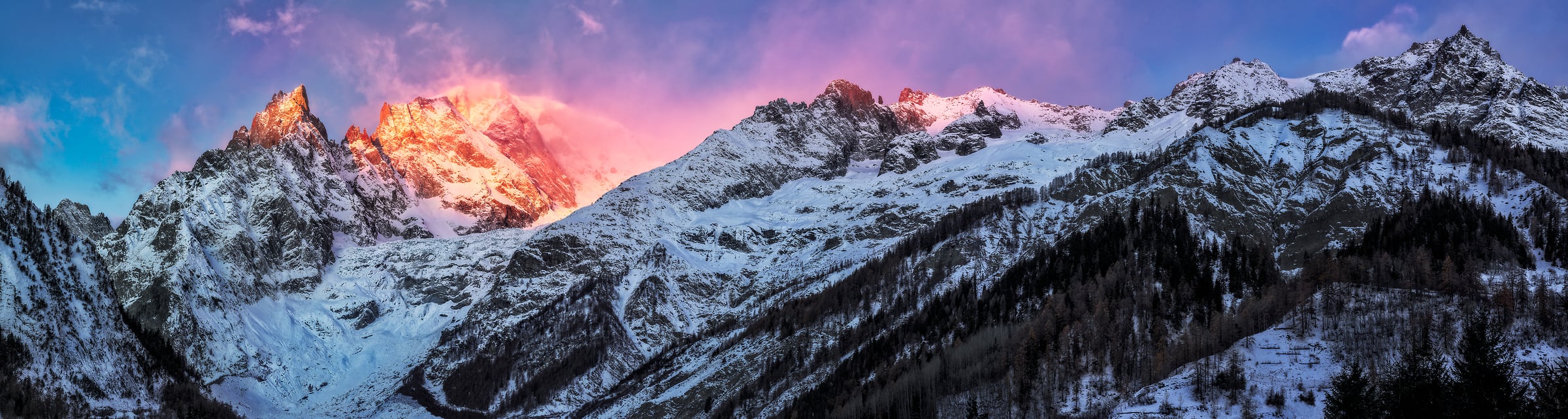This professionally-taken panoramic photo showcases a majestic mountainous landscape at either sunrise or sunset. The mountain range, primarily dark gray and black with sparse patches of white snow, displays a series of peaks and valleys with striking triangular points. On the right side, dense, dark green evergreen trees dot the sloping mountainside, whereas the left side is more curved and less forested. 

The sky is a mesmerizing blend of bright blue, orange, peach, purple, yellow, and red hues, with pinkish, misty clouds particularly evident on the left side, suggesting the sun's presence there. White clouds are scattered across the rest of the sky. The entire scene is bathed in a pink and yellow glow, casting a serene light over the landscape. The framing, focus, and lighting reflect a high level of professional skill, making this piece a perfect candidate for display in a home or museum, embodying natural beauty as art through photography.